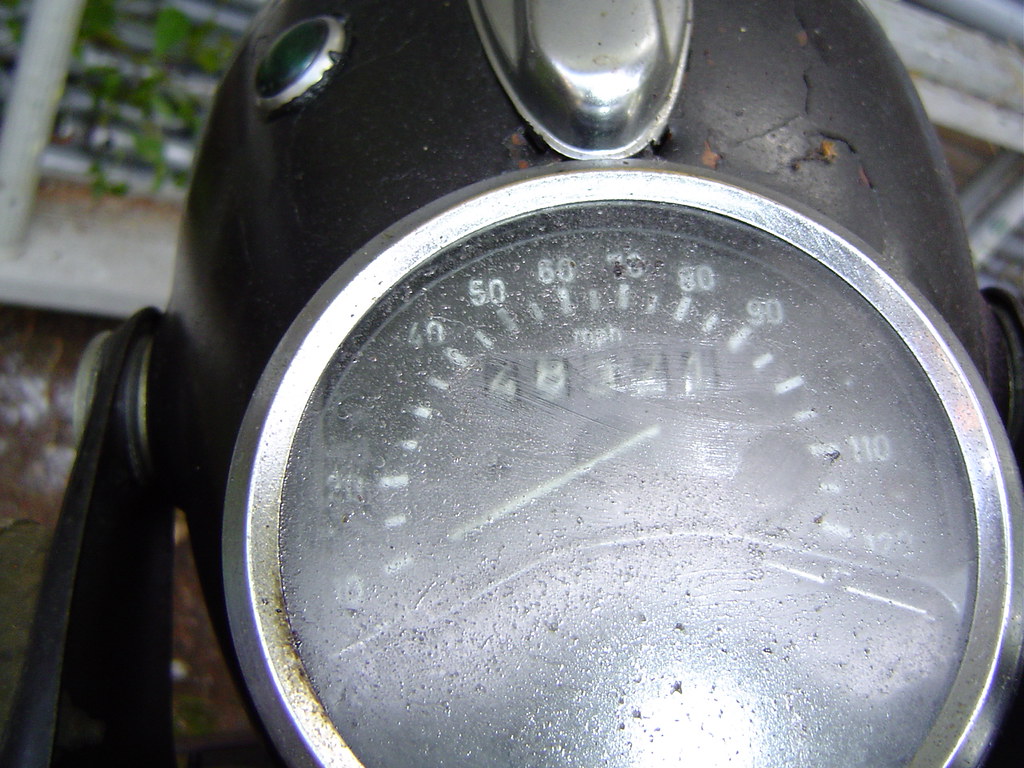The image captures a close-up view of a motorcycle gauge, prominently featured against the backdrop of a partly visible black gasoline tank. Central to the composition is a silver dial surrounded by a substantial, reflective silver bezel. The dial, encased in greasy and dusty glass, displays a speedometer reading from 0 to 120 MPH with an odometer reading of 48171 miles. A knob is positioned to the left of the gauge assembly. In the background, a white grate is interspersed with shrubbery, contrasting with the dirt-colored ground beneath. An arm is seen gripping the side of the tank on the left, while the gas tank itself shows signs of wear, including cracks, possible rust on the top right, and tarnish on the left side of the bezel. The light source, slightly off-center to the bottom right, creates reflective highlights on the dirty glass and the surrounding bezel.